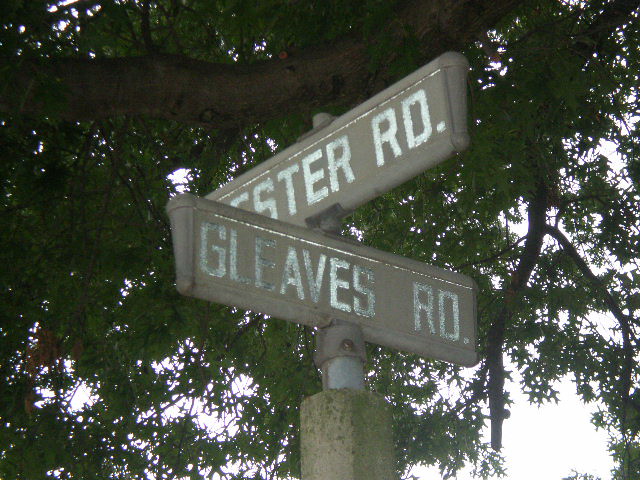A vintage street sign stands tall amidst a backdrop of leafy trees under an overcast sky. The dual-sign arrangement features a subdued beige-brown background with bold, white capitalized lettering. The top horizontal sign, partially readable, appears to indicate "Esther Road." Below it, the vertical sign distinctly reads "Gleaves Road" in crisp, white capitalized text. Both signs are mounted on a slender, silver metal post anchored by a concrete base. The muted colors of the sign and the soft blue light of the cloudy day create a calm and slightly nostalgic atmosphere.